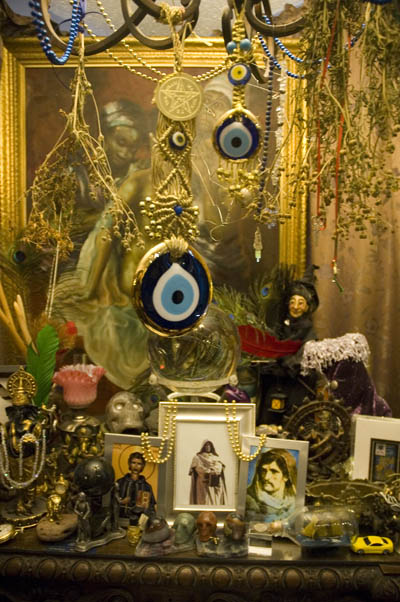The image depicts a meticulously arranged religious shrine adorned with various symbolic elements. Dominating the top portion, clusters of dried, withered greenery resembling sage hang in muted shades of light green, contributing to a sense of reverence and antiquity. Intertwined among the foliage are several strands of beads and necklaces. These adornments include a striking combination of blue beads on the left, a golden strand in the center, and another blue strand on the right, harmonizing with the natural dried elements.

Central to the shrine are circular symbols, intricately designed with gold perimeters and blue accents, featuring eye-like motifs with white sclera, blue irises, and black pupils. These symbols, possibly protective or warding in nature, hang gracefully among the bead strands. Above this array, a golden circular pentagram stands prominently, adding to the mystical aura of the shrine.

Beneath these hangings, an assortment of photographs showcases revered religious figures, their images bordered with silver trims, offering a visual homage to faith and spirituality. Interspersed with the photos are statuettes, some depicting skull-like figures, enhancing the eclectic and ritualistic feel of the shrine. Each photograph is meticulously draped with additional beads, creating a multi-layered tableau of devotion.

In the background, a Renaissance-style painting captures the visage of a black woman, complete with a headband, nestled among the spiritual paraphernalia. This adds a historical and cultural depth to the scene. Curiously, the bottom right corner of the image features a small, yellow car, contrasting sharply with the shrine's otherwise sacred and timeless ambiance, introducing an intriguing element of modernity amidst the traditional setup.